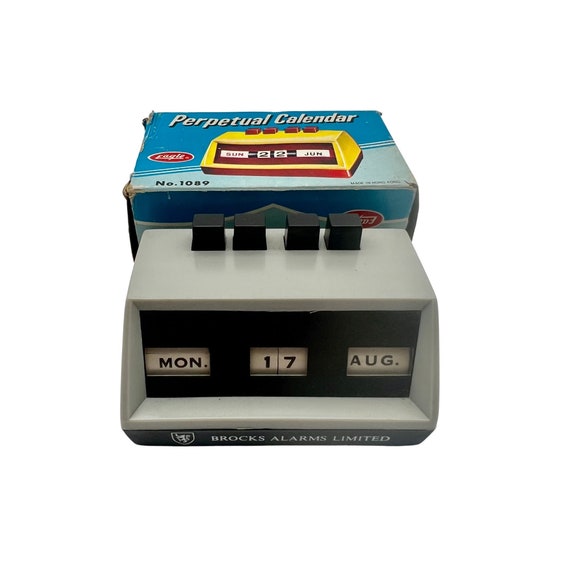This is a detailed photograph of a vintage electronic device, specifically a perpetual calendar. The device, positioned in front of its original packaging, is a roughly rectangular, light gray plastic object. On the front of the device, a recessed black screen prominently displays the day and date with three white rectangular windows arranged in a row. These windows read "MON," the date "17," and "AUG," respectively, all set against a black background. A strip of black runs along the bottom of the front panel, displaying the brand name "Brock's Alarms Limited" in white text. 

At the top of the device are four black square buttons, which are likely used to adjust the displayed date. The calendar functions through manual adjustment rather than digital means, signifying its vintage nature.

Behind the device sits its original box, which appears slightly worn around the edges, lending to its vintage aesthetic. The box is primarily dark blue, accentuated by lighter blue shades and diagonal stripes. It features an image of the same calendar in a yellow plastic version with red buttons, along with black numbering, suggesting variations in the product line. The box also highlights the product name "Perpetual Calendar" in white font. A red symbol with illegible white text is present, and a text number "1089" can be seen towards the bottom of the box. This image beautifully captures the nostalgic charm of the perpetual calendar, showcasing both the device and its packaging with great detail.